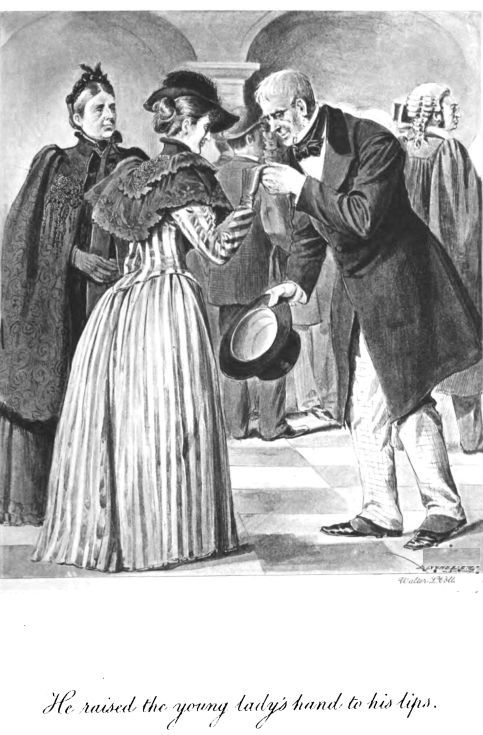The image is a detailed, vintage black-and-white illustration, likely from the turn of the century. It shows an older, formally-dressed man with short white hair, wearing a long coat adorned with fur around the collar and holding a black top hat in his right hand. He is bowing slightly to kiss the hand of a young lady. The man is attired in light-colored pants, a white shirt, black bow tie, and black shoes. The young lady, positioned on the left, wears a large black hat, her curly hair tied back, and a leather glove on her raised hand. She is draped in a shawl and donned in a long, elaborate dress that features vertical gray stripes on its wide skirt. Beside her stands an older woman, possibly her mother, dressed in a knee-length fur coat over a dark skirt, her hair pulled back and topped with a hat. The scene is framed by the cursive text at the bottom, which reads, "He raised the young lady's hand to his lips."